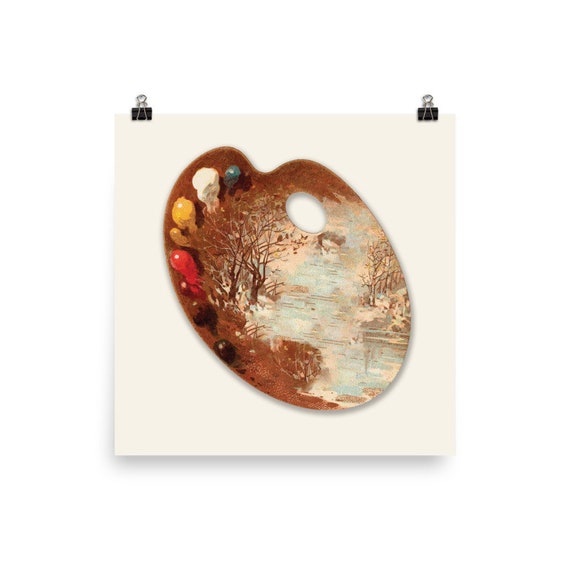The image depicts a unique art piece drawn on a square white sheet of paper, held up by two silver and black clips at the top corners. The artwork features a painter's wooden palette, characterized by its distinctive oval shape with a thumb hole. The palette is adorned with an array of paint splotches in various colors: dark green, white, goldish yellow, red, brown, and black. Central to the palette is an intricate painting of a nature scene. The scene prominently features a brown coastline with trees, which display branches and trunks in shades of brown and gray. A serene lake runs between two embankments, depicted with pale blue water accented by white lines. On the left, a cluster of trees stands out against the predominantly brown landscape, while the right side hints at another tree and additional brush. The detailed composition may suggest the presence of a small, indistinct figure in the water, adding a subtle touch of mystery to the scene. The entire artwork is presented against a transparent background, emphasizing its delicate and elaborate design.